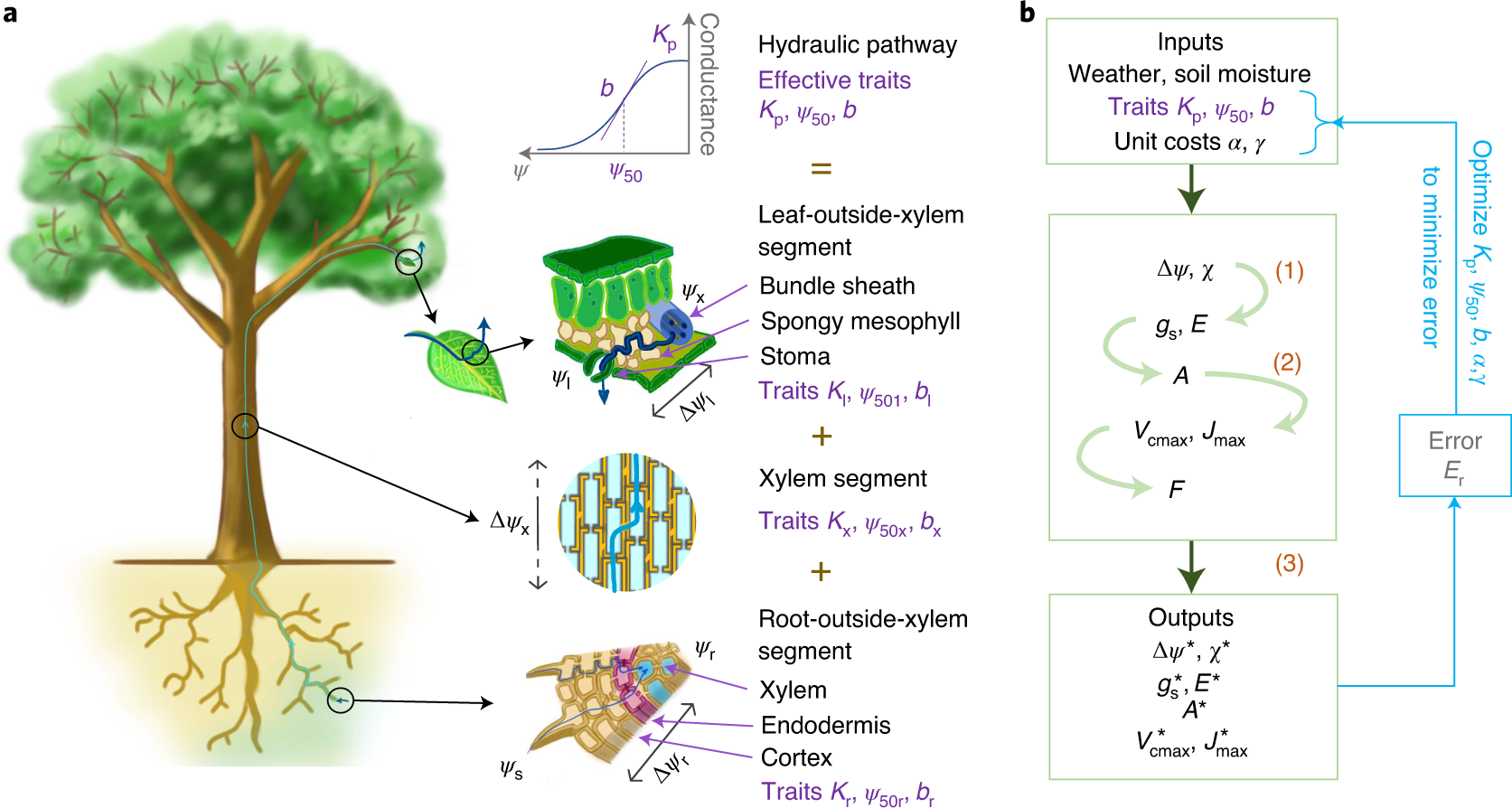The image is a highly detailed and technical diagram likely sourced from a textbook or a slide presentation aimed at engineers working with water systems. On the left-hand side of the image, there is an illustration of a tree, complete with green leaves, brown branches, and visible roots extending into the ground. This schematic is divided into two main sections labeled A and B.

**Section A** focuses on the biological and hydraulic processes within the tree. It begins with a "hydraulic pathway," detailing various components from the top down, including "effective traits" and their corresponding formulas. Key terms and diagrams highlighted in this section include:

- "Leaf outside xylem segment" with an illustration indicating the bundled sheath and spongy mesophyll.
- "Xylem segment" with explanations and associated formulas.
- "Root outside xylem segment," with a diagram showing the xylem, endodermis, and cortex, complemented by another set of formulas.

Arrows guide the viewer from the tree illustration to various parts of the detailed schematics that explain how water moves through the tree's anatomy, indicating processes related to photosynthesis and water transport.

**Section B** delves into external factors affecting tree growth and water transport, marked by inputs and outputs with various equations. The uppermost part of this section mentions inputs such as "weather" and "soil moisture," followed by unit costs, each illustrated with formulas in green-bordered boxes. The section shows a progression from inputs to a series of intricate calculations, eventually leading to outputs. These outputs are also encapsulated within green-bordered boxes, with an overarching focus on optimizing and minimizing error, represented visually with arrows and formulas.

The overall composition is presented on a white background, combining diagrams, text, and calculations in black lettering, making it a very complex and informative piece that would require careful analysis to fully understand.